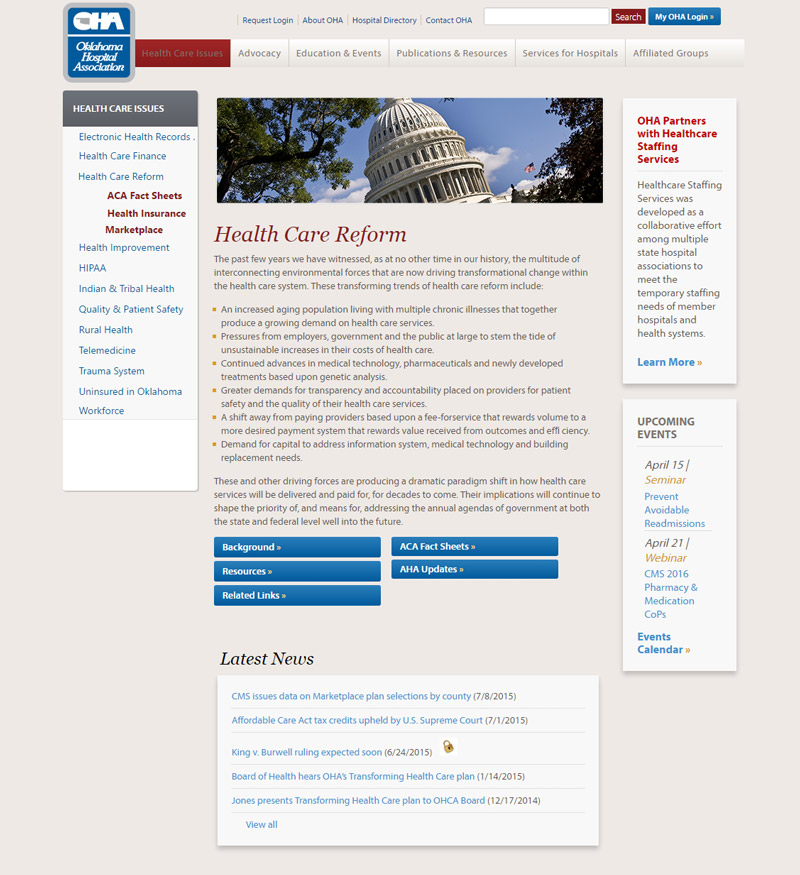In this image, we see a screenshot of a website belonging to the Oklahoma Hospital Association (OHA). The upper left corner features a blue box containing the OHA logo, with the full name, "Oklahoma Hospital Association," displayed beneath it. Below the logo is a navigation bar with a gray background labeled "Healthcare Issues," presenting an organized list of links for various topics. 

The topics are divided into sections by color. The first set, in a gray font, includes "Public Health Records," "Healthcare Finance," and "Healthcare Reform." The next section, in red text, features "ACA Fact Sheets" and "Health Insurance Marketplace." Following that, in blue text, we see links to "Health Improvement," "HIPAA," "Indian and Tribal Health," "Quality and Patient Safety," "Rural Health," "Telemedicine," "Trauma System," "Uninsured in Oklahoma," and "Workforce."

At the bottom of the page is a white box titled "Latest News." Within this section, two news headlines are displayed: "CMS issues data on Marketplace plan selections by county 7-8-2015" and "Affordable Care Act Tax Credits, upheld by U.S. Supreme Court."